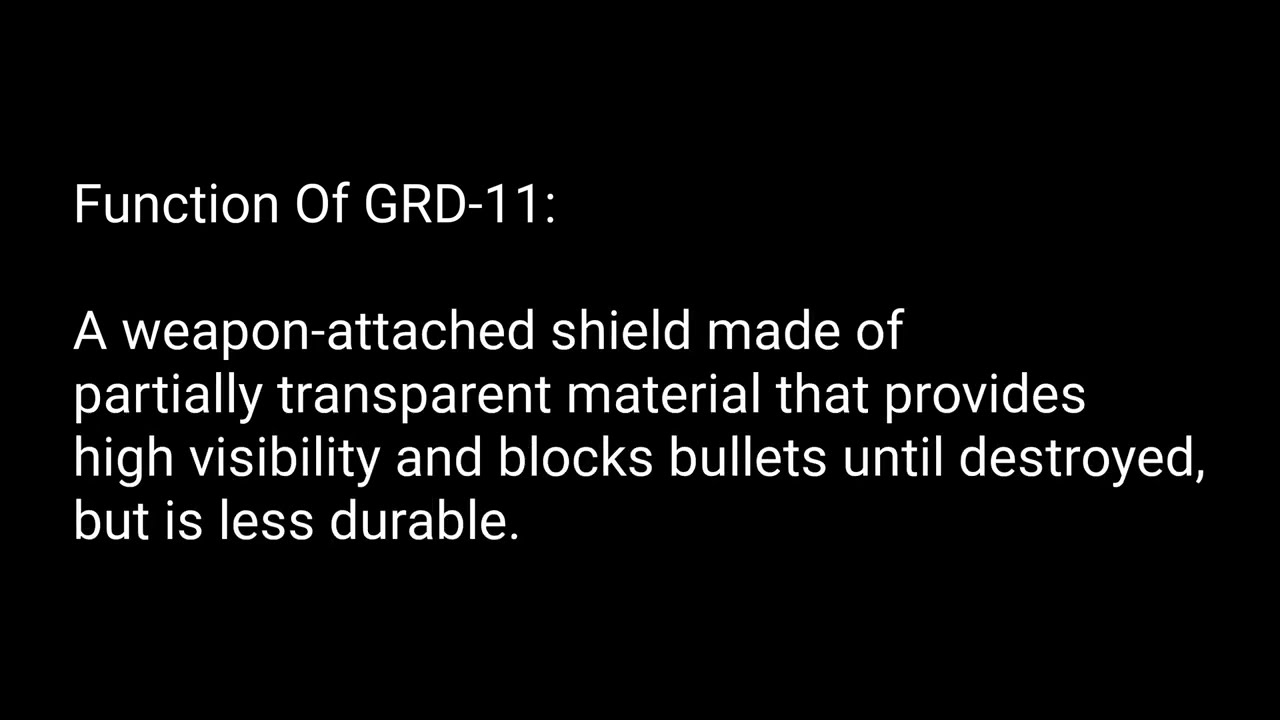The image presents a simple, text-based slide with a black background and plain white text. The text explains the function of "GRD-11" and reads: "Function of GRD-11: A weapon-attached shield made of partially transparent material that provides high visibility and blocks bullets until destroyed, but is less durable." There are no objects or additional visuals in the image; it is purely focused on the detailed description of the GRD-11 shield's capabilities and characteristics.